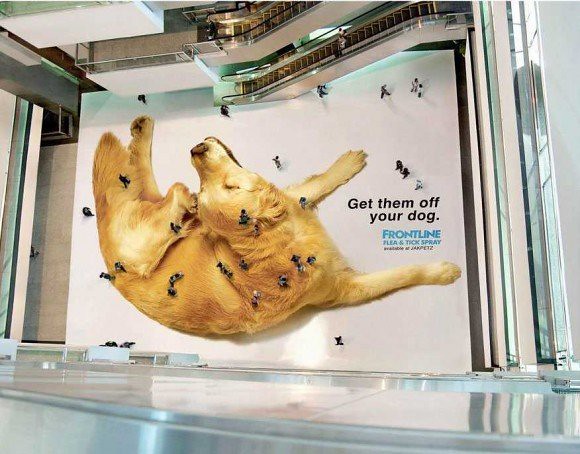This clever advertisement, located on the bottom floor of a multi-story mall, spans a significant portion of the floor space. The ad features an image of a blonde golden retriever Labrador mix scratching its head with its back paw. The photo was taken from a vantage point at least three or four stories above, looking directly down at the floor. Due to the constant flow of mall-goers walking across the advertisement, the people appear as if they are fleas on the dog. To the right of the dog, the text reads, "Get them off your dog," promoting Frontline Flea and Tick Spray. This creative placement combines visual illusion with effective marketing to catch the attention of shoppers.